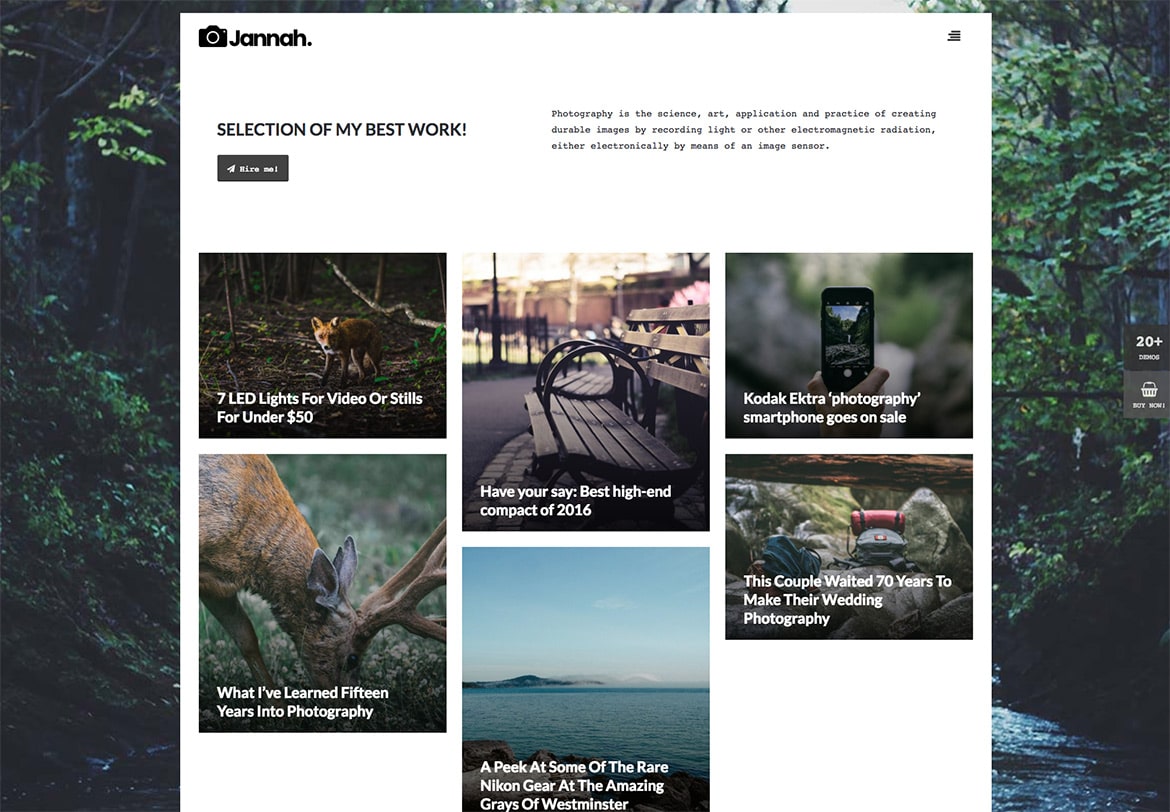The website's homepage is visually set against a lush forest landscape bordering a tranquil river, surrounded by verdant greenery and towering trees. Atop this serene background sits a stark white square, prominently displaying the site's key elements. 

On the right side of this square, the website's name "JANA" is emblazoned beside a minimalistic camera icon, signifying its focus on photography. Just below this header, a tagline reads "Selection of My Best Work," hinting at a curated gallery of the creator's top photographic pieces.

To the left, there's an informative block of text detailing the essence of photography, describing it as "the science, art, and application, and practice of creating durable images by recording light or other electromagnetic radiation, either electronically or by means of an image sensor."

Beneath this textual content, a series of five images is arranged in a row, each serving as a visual link to separate articles. While the image titles indicate clickable content, they collectively promise a deeper exploration into the world of photography through the lens of the artist.